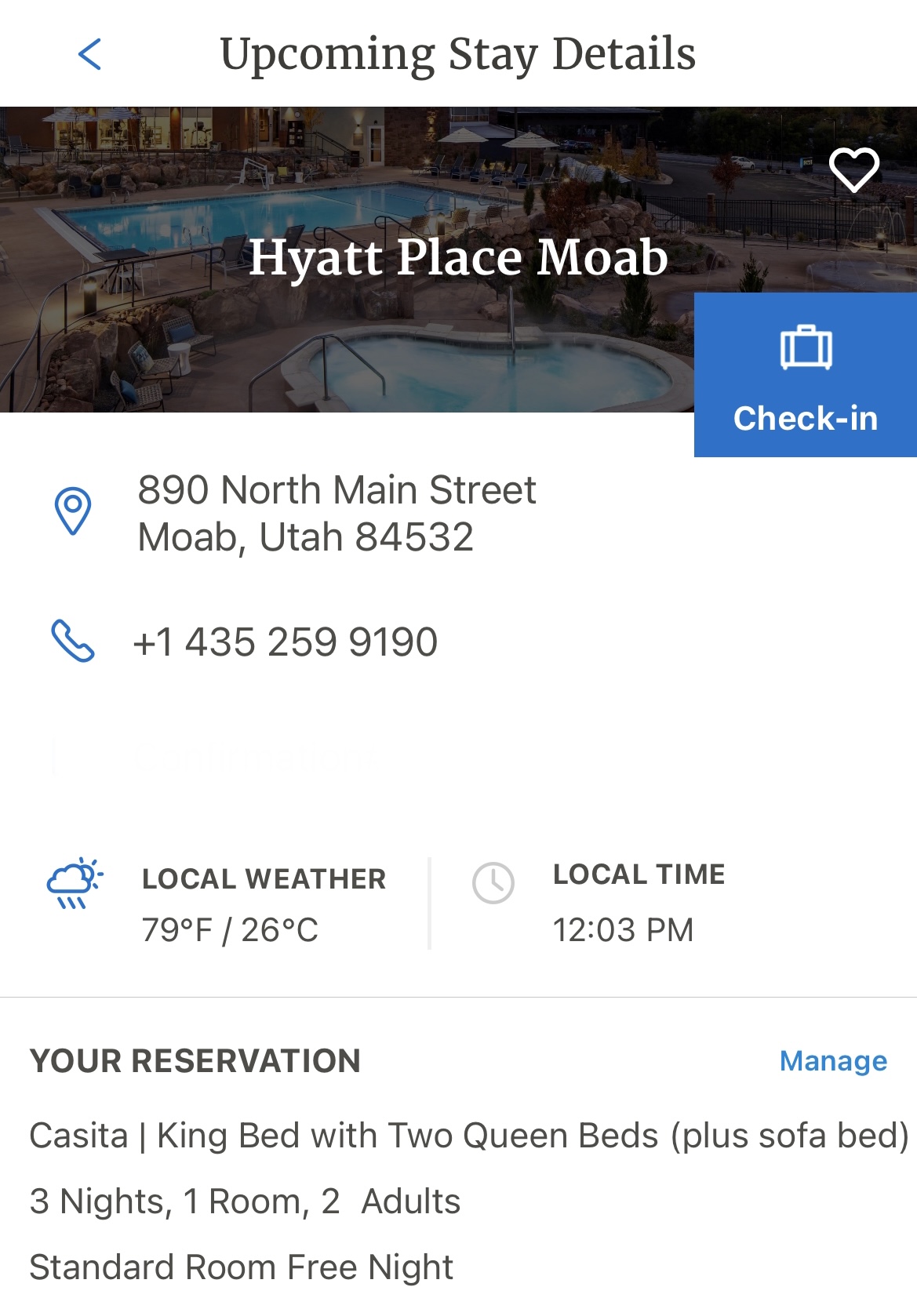Screenshot of hotel reservation details displayed on a mobile device. At the top, the header reads "Upcoming Stay Details" with a left-pointing caret. Below the header, there's a small thumbnail image of Hyatt Place Moab. The image depicts the exterior of the hotel, showcasing two swimming pools: one long and rectangular with blue water, and the other heart-shaped with a lighter blue hue. Surrounding the pools are multiple lounge chairs and two umbrellas. The image has a dark overlay, and over it, the words "Hyatt Place Moab" appear in white, with a heart icon in the upper right corner.

In the background of the image, there is a building with numerous windows and a visible fountain. Adjacent to the thumbnail, a small blue square icon indicates "Check-in" with a suitcase symbol. Directly below, a Google Maps location tab specifies the address: "890 North Main Street, Moab, Utah, 84532." Additionally, there is a telephone icon with the number "+1 435-259-9190."

Further details include a small cloud icon with the sun and raindrops, showing the local weather as 79°F (26°C). To the right of the weather, a clock face icon displays the local time as 12:03 PM. Following these details, the text "Your Reservation" appears, with a blue "Manage" button on the right.

In the reservation summary, it lists: "Casita King Bed with Two Queen Beds + Sofa Bed." Below this section, it specifies: "Three nights, one room, two adults, standard room, free night."

This thoroughly detailed caption encapsulates the essence of the screenshot, providing clarity and specificity for all visible elements.